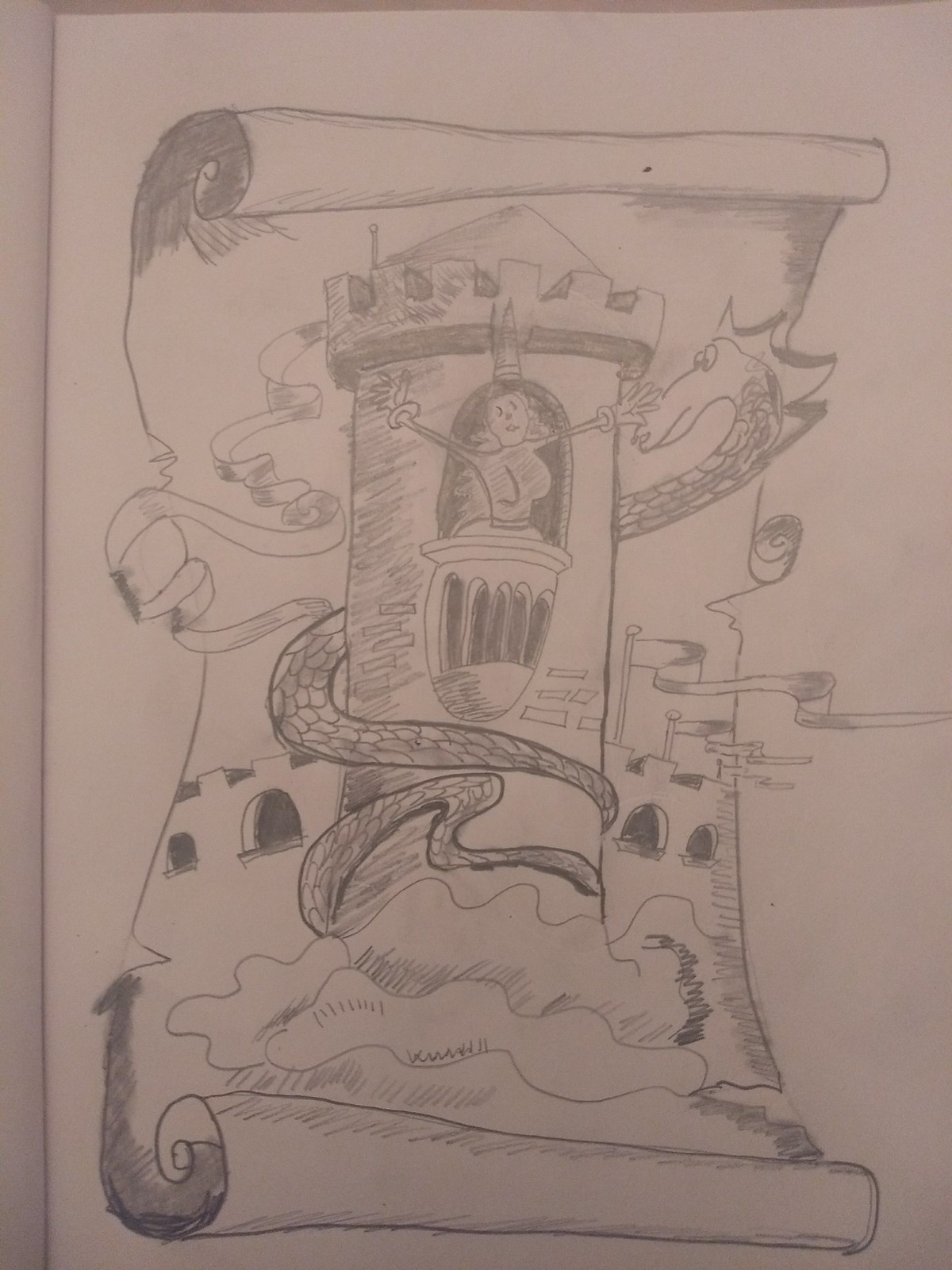The image depicts a meticulously crafted pencil drawing on white paper with a vintage scroll as the backdrop. The scroll's edges are artistically torn, and both the top and bottom are elegantly rolled up, exuding an ancient, timeworn appearance. At the heart of the scroll lies a cartoonish castle tower, extending vertically. A princess, arms spread open, leans out of a window near the top of the tower, creating a focal point for the viewer. 

Encircling the tower is a colossal, serpentine dragon, coiling its immense body around the structure. The dragon's head emerges menacingly on the right side, its gaze fixated intently on the princess. Below the tower, the castle's lower sections are depicted with detailed walls adorned with open windows, fluttering flags, and ornate banners. The very base of the scroll reveals a grassy ground, grounding the fantastical scene. The entire illustration remains a monochromatic masterpiece, emphasizing the intricate pencil work and the enchanting narrative it portrays.